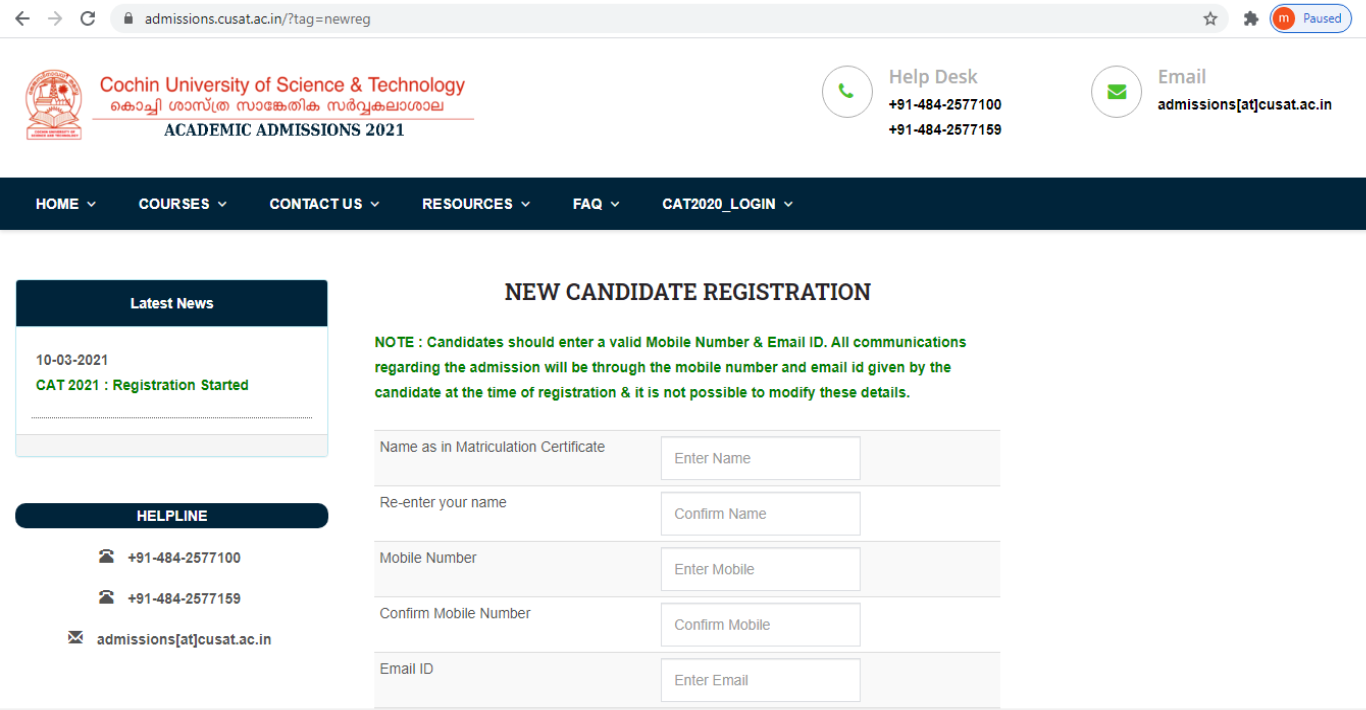Screenshot from the Cochin University of Science and Technology (CUSAT) Academic Admissions 2021 webpage, hosted on admissions.cusat.ac.in. 

In the upper left corner, there is a prominent red seal, representing the university's emblem. The upper right corner features contact information icons: a green phone symbol and a green envelope, each within distinct circles. Adjacent to these symbols, the text "Help Desk" is displayed, along with the contact numbers: +91 484 2577100 and +91 484 2577159. Additionally, the email address provided is admissions@cusat.ac.in for further inquiries.

Below the header, a navy blue navigation bar includes links to Home, Courses, Contact Us, Resources, FAQs, and CAT 2020 Login.

The main body of the page is dedicated to the "New Candidate Registration Form." Notably, it includes a cautionary note in green font: "Candidates should enter a valid mobile number and email ID. All communications regarding the admissions will be through the mobile number and email ID given by the candidate at the time of registration. It is not possible to modify these details." 

The page also contains various input fields for candidates to provide their necessary information for registration.